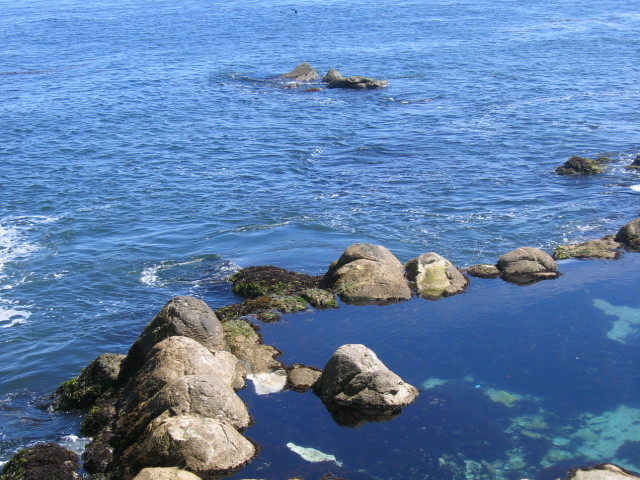The photograph captures a serene coastal scene dominated by blue ocean waves contrasting with rocky outcrops. The foreground features a circular arrangement of large, grey, and black rocks forming a natural tide pool with calm, still water. This tide pool's surface is tinged with moss and algae, suggesting a tranquil, self-contained ecosystem. In stark contrast, the surrounding ocean water is active, characterized by light aqua blue waves and ripples edged with white foam, indicating movement and vibrancy. Further out, additional rocks punctuate the horizon, emphasizing the rocky nature of the shoreline. The sky, though not clearly depicted, hints at clear, sunny conditions, evidenced by the vivid illumination and clarity of the photograph. No text, people, or specific location details are present.